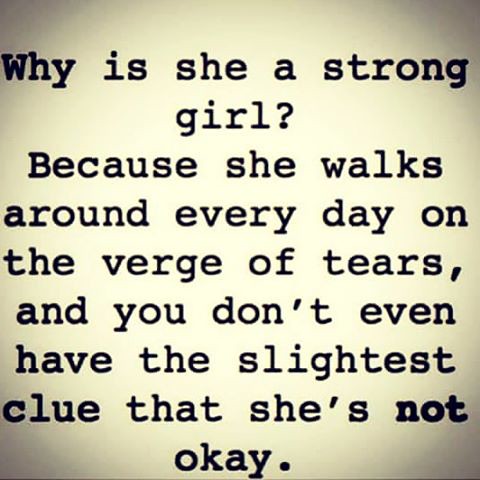The image depicts a meme or social media message featuring black typewriter-style text on an off-white, almost beige background. The text, centered and taking up most of the image, reads, "Why is she a strong girl? Because she walks around every day on the verge of tears, and you don't even have the slightest clue that she's not okay." The phrase "Why is she a strong girl?" stands out on its own line, and the words "girl" and "okay" are prominently centered rather than left-aligned. The borders of the image have subtle darker gray shades extending from the corners, adding some depth to the otherwise minimalistic design.